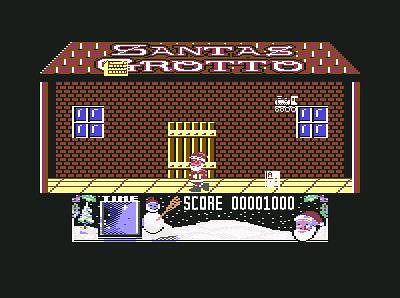In this still from an unidentified video game, the focal point is a brick building showcased against a stark black background, predominantly featuring shades of brown. Santa Claus is seen walking on a distinct yellow sidewalk in front of the building. At the rooftop of this structure, there is a sign that reads "Santa's Grotto," indicating a festive theme. The building itself is detailed with two windows and a uniquely designed door that resembles a fence. Below the building, game elements are displayed, including the word "Score" followed by a numeric value of 1000, alongside Santa's face, possibly tracking the player's progress or points. The scene is set in a snowy landscape with a snowbank visible, where a snowman stands adding to the wintery ambiance. Additionally, some text or icons, perhaps representing the time or another game mechanic, appear towards the bottom of the image, though it is partially obscured. Santa's journey across the sidewalk suggests he is en route to new adventures beyond this scene.